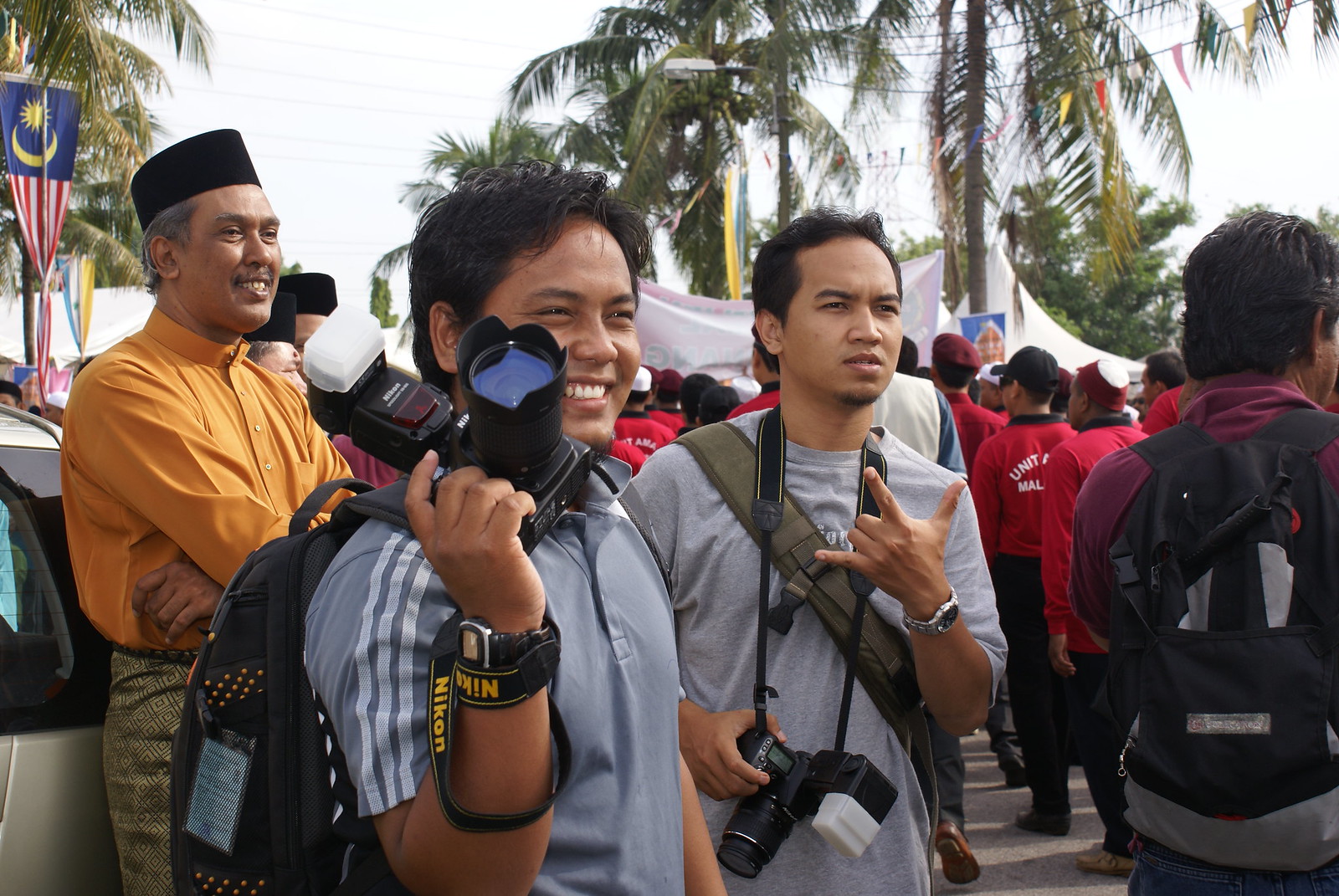In this detailed outdoor photograph, taken during the day, two Asian men prominently stand amidst a bustling crowd. Each man is holding a camera, hinting at an event possibly attracting photographers and journalists. The man on the left is smiling and is dressed in a gray shirt with white stripes, a wristwatch, and the word "Nikon" visible on his camera strap. His companion, also sporting a wristwatch, is captured in action with a camera held close. The vibrant setting features various onlookers, including several men in red jackets or shirts, one of whom dons a black baseball cap, all seemingly focused on an unseen event to the left. Behind the two main subjects, another Asian man in a yellow shirt and black hat stands out. The scene is framed by a gray sky, festive triangular banners strung from palm trees, and a distinctive flag showing red and white stripes, a blue field, and a yellow crescent. On the right, partially turned away from the camera, a man with long black hair carries a gray backpack. Farther left, another individual in an orange shirt and hat leans casually against a car, adding to the dynamic yet harmonious composition of the scene.